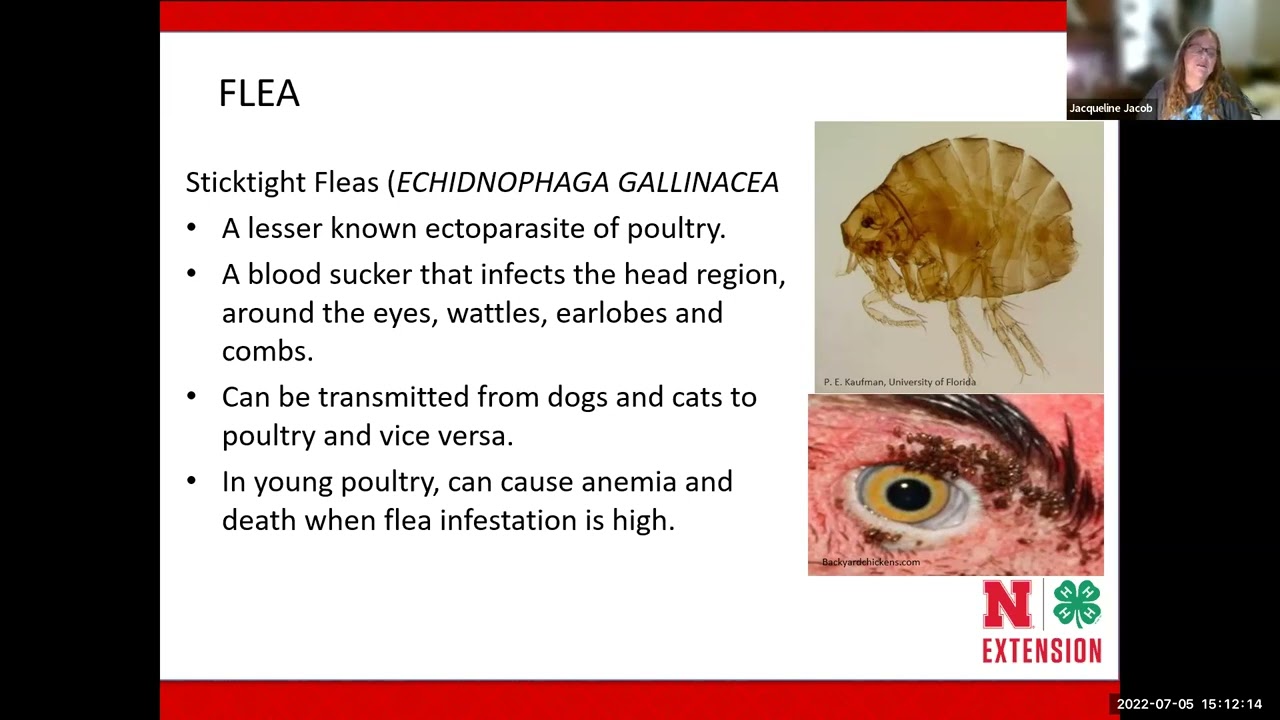The image appears to be a screenshot from a Zoom call featuring a slide on flea information, presented by Jacqueline Jacob, whose webcam appears in the top right corner showing her blurred background and long hair. The slide, with a black background and bordered in red, is titled "Flea" and highlights the stick-tight flea, a lesser-known parasite of poultry. It describes how these blood-sucking ectoparasites affect the head region around the eyes, wattles, earlobes, and combs, and can be transmitted between dogs, cats, and poultry, potentially causing anemia and death in heavily infested young poultry. Accompanying the text are two images: a highly magnified flea and a close-up, distressing photo of a chicken's eye infested with fleas. The slide's specific date is July 5th, 2022.